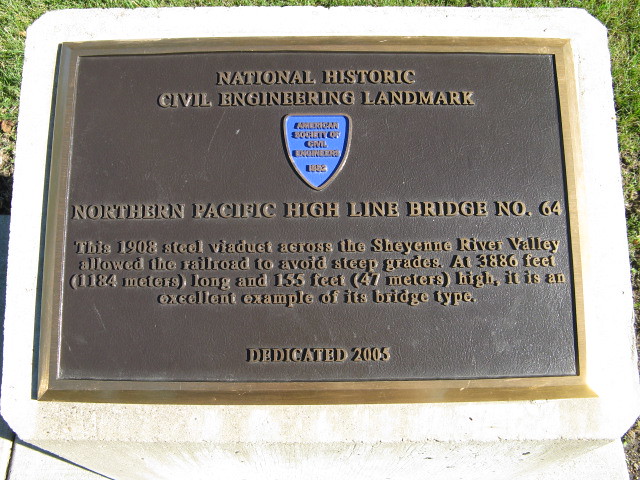The plaque, situated outdoors against a backdrop of green grass, is a cement memorial with a bronzed inlay, dedicated as a National Historic Civil Engineering Landmark. At the top, it reads "National Historic Civil Engineering Landmark," followed by a blue triangle emblem from the American Society of Civil Engineering, though its small lettering is hard to discern. Beneath the emblem, the plaque commemorates the Northern Pacific Highline Bridge No. 64. This 1908 steel viaduct, spanning 3,886 feet in length and standing 155 feet high, enabled the railroad to traverse the Cheyenne River Valley without encountering steep grades, exemplifying engineering excellence of its type. The plaque indicates that the bridge was dedicated in 2005.